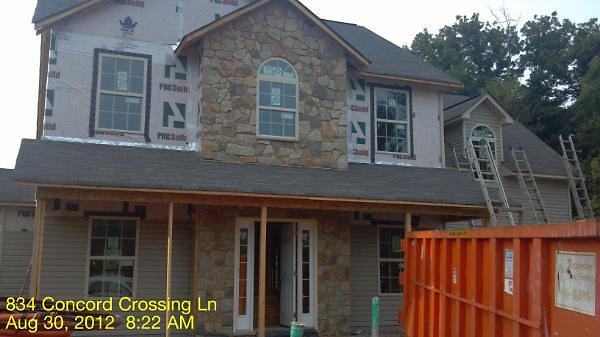The photograph captures an outdoor scene in front of a two-story house undergoing renovation. The house, located at 834 Concord Crossing Ln, is pictured on August 30, 2012, at 8:22 AM, as noted in yellow text in the bottom left corner. Dominating the foreground is an orange construction dumpster parked on the driveway. The house features a blend of architectural elements, most notably a central stone tower with an arched window adorned with glass panes. This tower extends from a ground-level white door, flanked by windows, up to the second story.

The house has a gabled roof design and a sizable porch supported by brown timbers, suggesting temporary structural support during the renovation. Several ladders—three prominently leaning against the house on the right side—indicate ongoing construction work. There's clear evidence of remodeling, with siding removed from the upper level and partially from the lower level, exposing some Teflon covering with construction-related text. Additionally, new windows have been installed, recognizable by the stickers still attached to the panes.

Temporary plastic sheets bearing the construction company's logo are also visible on the exterior, and various pieces of paper, likely construction notices, are taped to the windows. A tree in the background and the hint of a garage to the right of the frame complete the setting of this active renovation site.